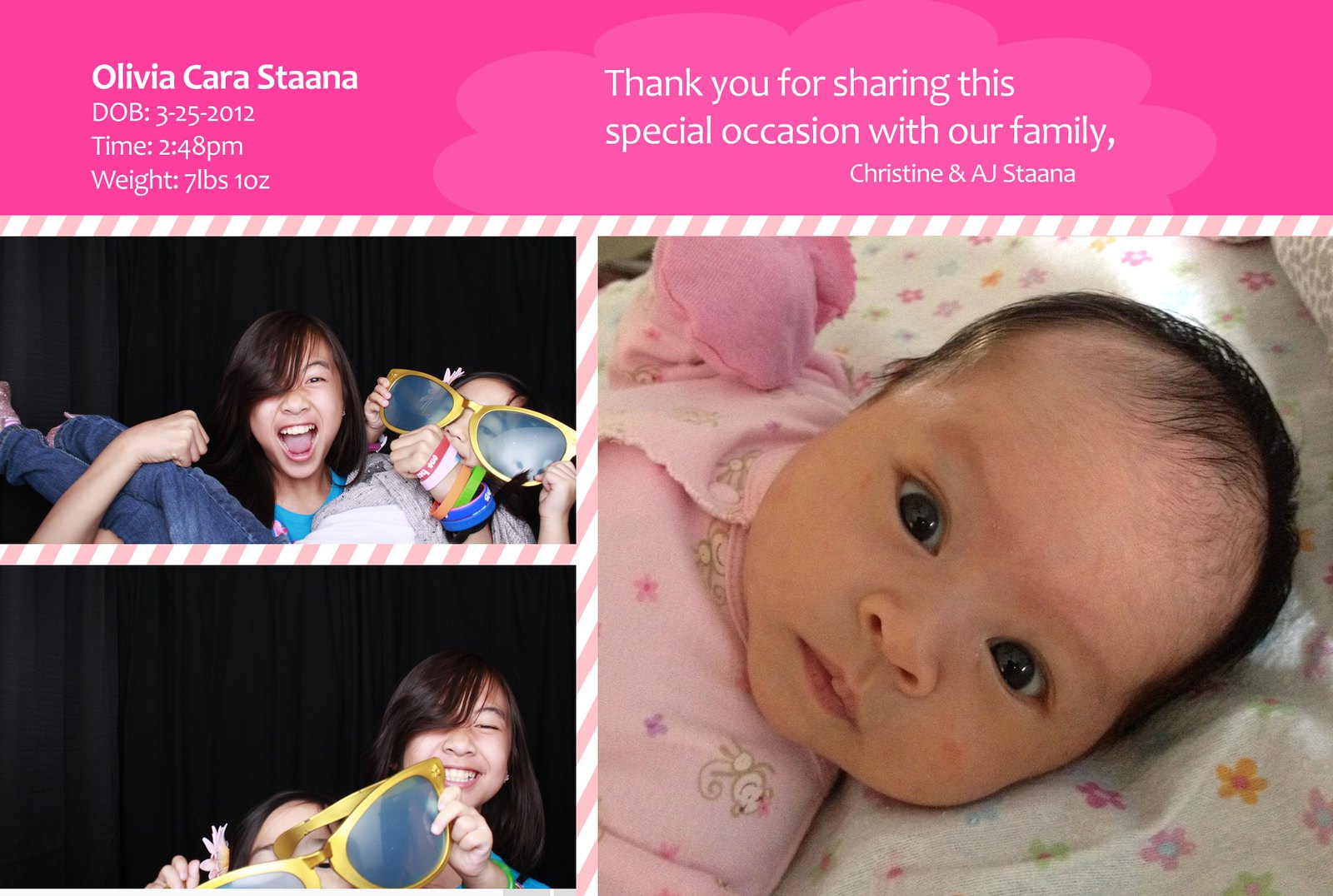The image is a collage centered around a touching family moment. The main focus is a large photo on the right, featuring a baby girl dressed in a pink outfit adorned with little cartoon monkeys, lying on a white mattress with flowers. She gazes into the camera with big brown eyes. On the left are two smaller photos, capturing a young girl holding the same baby at slightly different times, about five seconds apart. In these photos, the baby sports oversized golden sunglasses while the young girl, adorned with many wristbands on her left arm, cradles her gently. In the second smaller photo, the girl has let go, allowing the baby to stand on her own while still wearing the sunglasses. At the top of the collage, the text reads "Olivia Karasdena," along with the date of birth, time of birth, and weight of the baby. To the right, a heartfelt message says, "Thank you for sharing this special occasion with our family," signed by Christine and H.A. Stana.